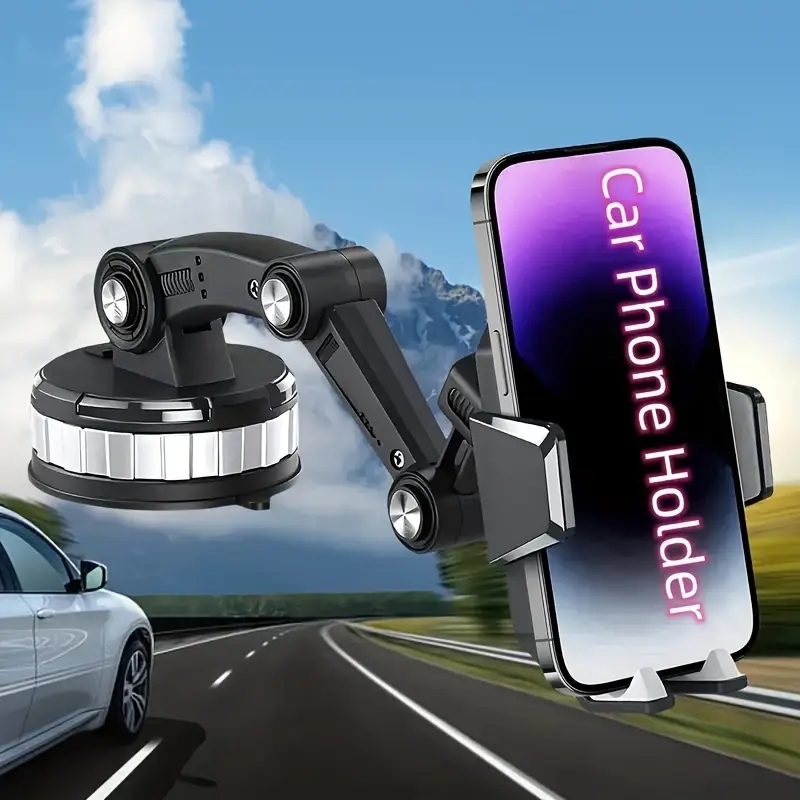The image is an animated advertisement showcasing a car phone holder. The background features a clear blue sky with a large, puffy white cloud to the left and a jagged, gray mountain partially visible on the right. At the center of the image is the car phone holder, which has a black circular base with silver rectangular segments in between. The holder features an extendable arm that bends at three points, each connected by a silver disc and visible screws. A demo phone, secured in the cradle, displays a screensaver with a gradient that transitions from purple at the top, blue in the middle, to white at the bottom. The text "Car Phone Holder" is prominently displayed on the phone screen in white letters edged in purple. In the lower left corner of the image, a white passenger car is seen driving down a dark black roadway.